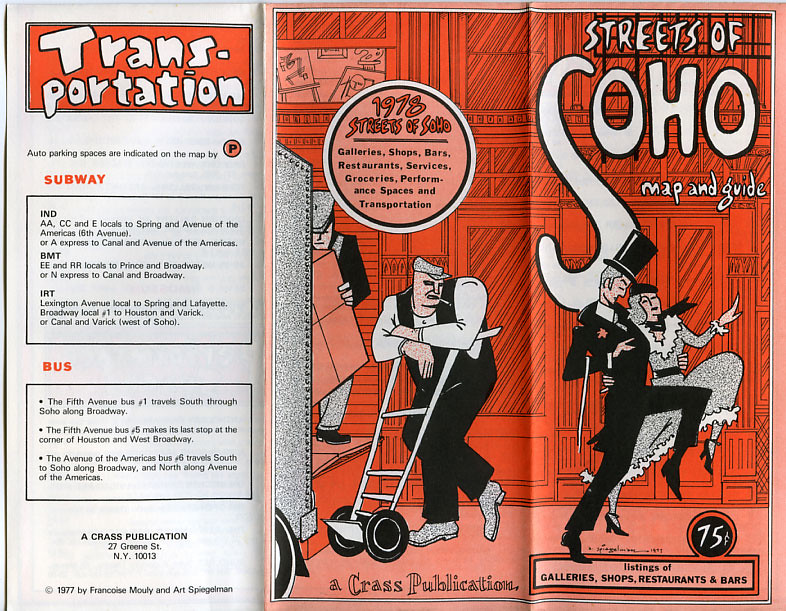This brochure, titled "Streets of Soho Map and Guide," features a vibrant cover with a man in a top hat and a woman in a dance dress and shoes, appearing to dance or walk together. Occupying two-thirds of the brochure, the main image also shows two men loading or unloading items from a truck. At the top, the title is prominently displayed. Below the image, the text states, "A Crass Publication," listing galleries, shops, restaurants, and bars, with a price tag of 75 cents. The left panel provides detailed transportation information, indicating that auto parking spaces are marked by 'P' on the map, and includes sections for subway routes and bus details, specifically noting the 5th Avenue bus that travels south through SoHo along Broadway. The bottom of the brochure is dated 1977 by Francois Moly and Art Spiegelman, with an address of 27 Green Street, New York, 10013. The reverse side reiterates the focus on galleries, shops, restaurants, services, groceries, performance spaces, and transportation, also marked as a publication from 1978.